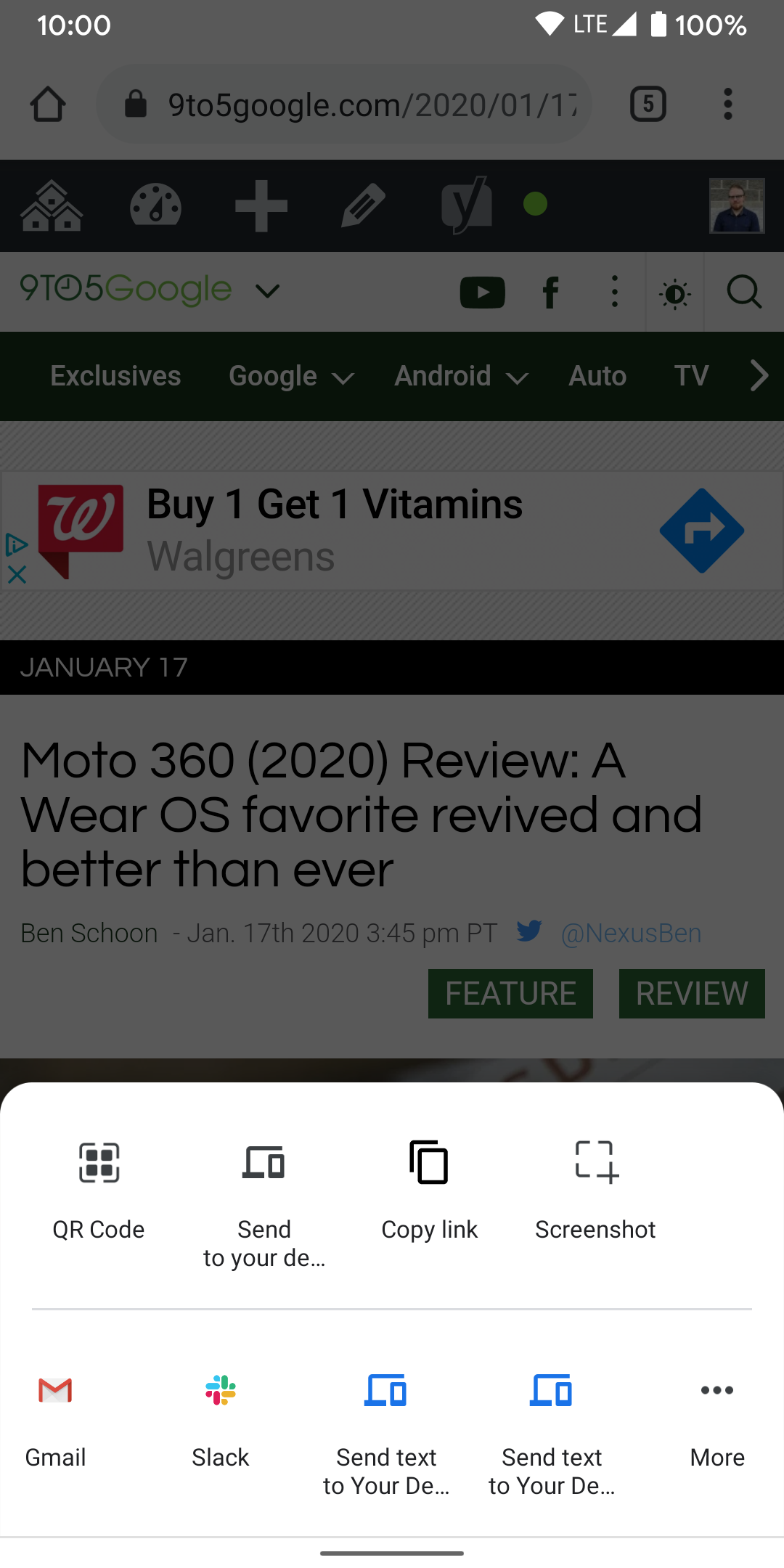The image showcases a dark-themed smartphone screen. The status bar at the top indicates it is 10 o'clock, with LTE connectivity, full signal strength, and a 100% battery level. The screen displays a webpage from '9 to 5 Google.' The header section is black, featuring tabs labeled 'Exclusives,' 'Google,' 'Android,' 'Auto,' 'TV,' and an arrow pointing to the right for navigation.

Beneath this, there is a white text box against a gray background advertising a Walgreens promotion: 'Buy One, Get One Free Vitamins.' Following this is a section highlighting a 'Moto 360 2020 Review,' described as 'A Wear OS Favorite Revived and Better Than Ever.'

Further down, there is a 'Feature Box' beside a 'Review' section. The background transitions to a bright white color, featuring icons for various actions: a QR code for device compatibility, options to send to your device, copy the link, take a screenshot, and share via Gmail or Slack. Additionally, there is an option to send a text message to your device, repeated twice, followed by three horizontal dots indicating more options.